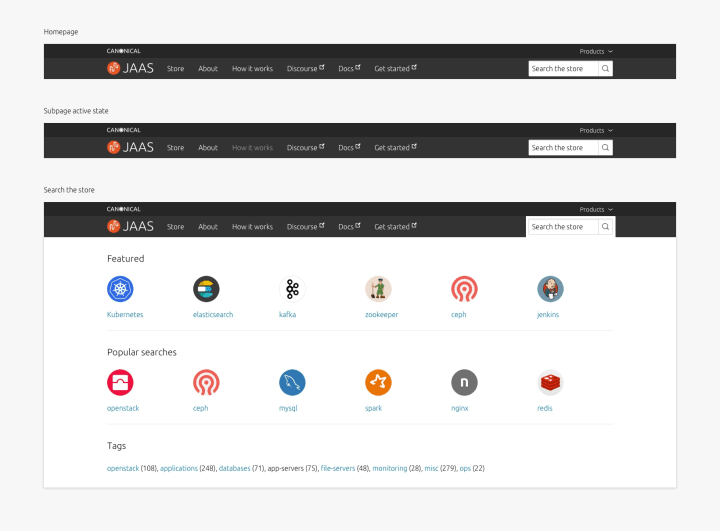The image showcases a detailed screenshot of a webpage with multiple navigation bars and sections. At the top of the screenshot, there is a primary navigation bar labeled "Homepage" and featuring various tabs such as "JAS," "More About," "How It Works," "Group Docs," "Get Started," and a search bar.

Below this main navigation, there is a repeated navigation bar which is slightly altered. This bar is marked "Sub Page, Active State" and appears to be an active sub-page. 

Further down, a third similar navigation bar reads "Search the Store." Beneath this bar, a section labeled "Featured" displays various logos and items, though the text is somewhat difficult to read. 

Some of the identifiable logos and text include:
- "Kilometers," which features indistinct text and graphics.
- A web symbol in a blue circle.
- "Electro," followed by an unclear word.
- "Kafka" with a molecule symbol.
- "Zookeeper," accompanied by an icon of a person holding a mop.
- "Seth," depicted with a red face in a circular design.
- "Jenkins," associated with a notable person icon.
  
On the right, under "Popular Searches," the following items are listed:
- "Open Stack," highlighted with an opening drawer icon.
- "Seth," repeating the previous red face symbol.
- "MySQL," illustrated with a hand in blue.
- "Bar," displaying an orange star.

The overall layout is structured with these repeated navigation elements and featured items, giving a comprehensive view of the webpage’s content and navigation structure.